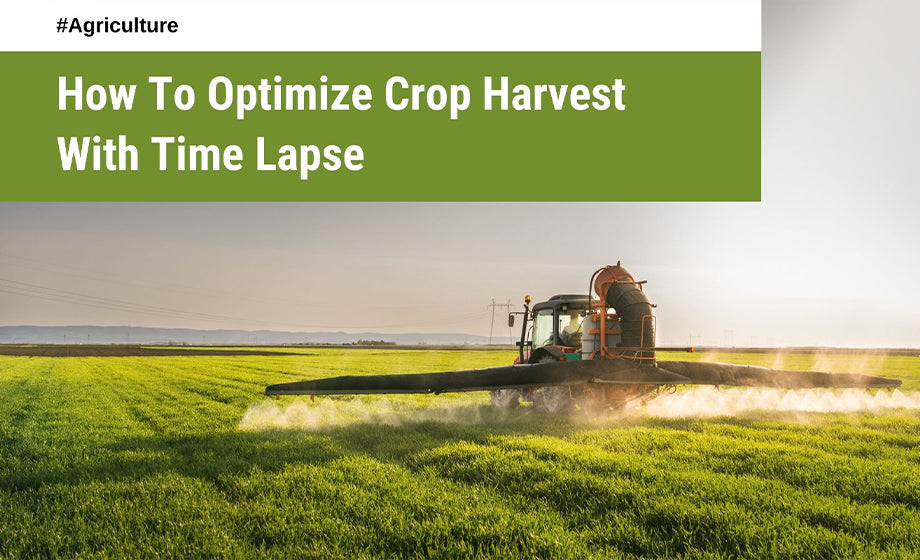The image depicts a vibrant, lush green farm field with an orange tractor-like farm vehicle prominently positioned in the lower right-hand side. The vehicle is equipped with a large, prominent fin or apparatus and a black tube extending upwards. It appears to be spraying a white mist, possibly chemicals or water, onto the field from its base. A man can be noticed operating the vehicle. In the background, the sky appears grey, with distant silhouettes of power lines and purple-tinged mountains. Overlaying the image are two rectangular text boxes in the upper left corner: a white box displaying "#agriculture" in black font, and a green box beneath it with the text "How to optimize crop harvest with time lapse" in white font, suggesting the image might be part of a presentation slide.